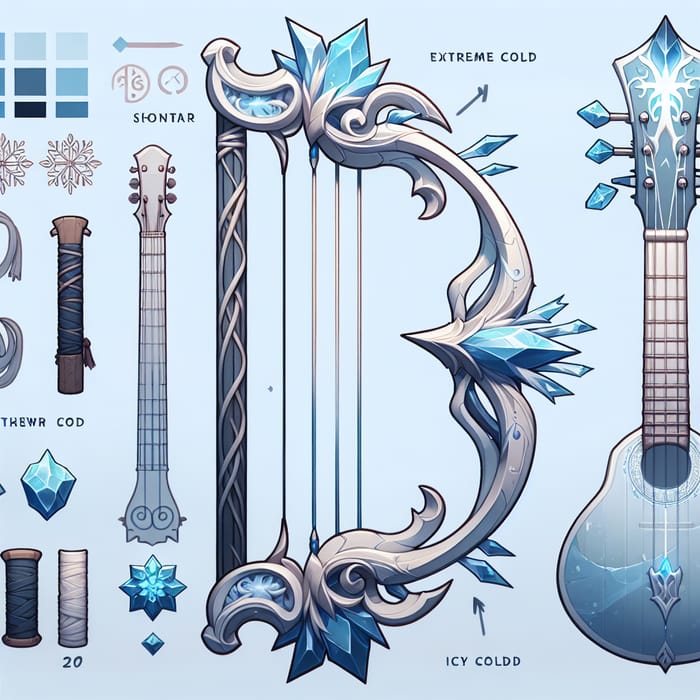This digital drawing illustrates a collection of intricately designed musical instruments set against a light blue background, emitting an icy, ethereal vibe. On the left, a series of blue and gray square designs transition into various symbols and floral motifs, suggesting intricate detailing and ornamentation. Below this ornate border, a mysterious tube-like instrument, partially obscured, displays the letters "T-H-E-W-R, COD" and is wrapped in what looks like twine, accompanied by an inscription with the number "20." A gem-like, blue diamond shape sits below these elements.

The center column features the label "Chanteur" and appears to depict the handle of a guitar with more of the distinctive blue diamond embellishments. Dominating the middle is a harp-like structure with a curved form, integrated blue highlights, and a pointed arrow indicating the icy blue gems. This component is labeled with the text "I-C-C-O-L-D-D," possibly alluding to its frosty aesthetic, with an additional label marking parts of the harp as "Extreme Cold."

To the right, another instrument resembling a guitar or mandolin showcases a predominantly blue coloration on its handle and base, adorned with similar blue crystal-like gems. This instrument, like its harp counterpart, is partially transparent, accentuating the ice-like material from which it's crafted. The visual presentation is not only artistic but also somewhat functional, as it breaks down the intricate parts and their icy textures, creating a cohesive and mesmerizing illustration of what seems like fantastical, vintage musical instruments forged from ice.